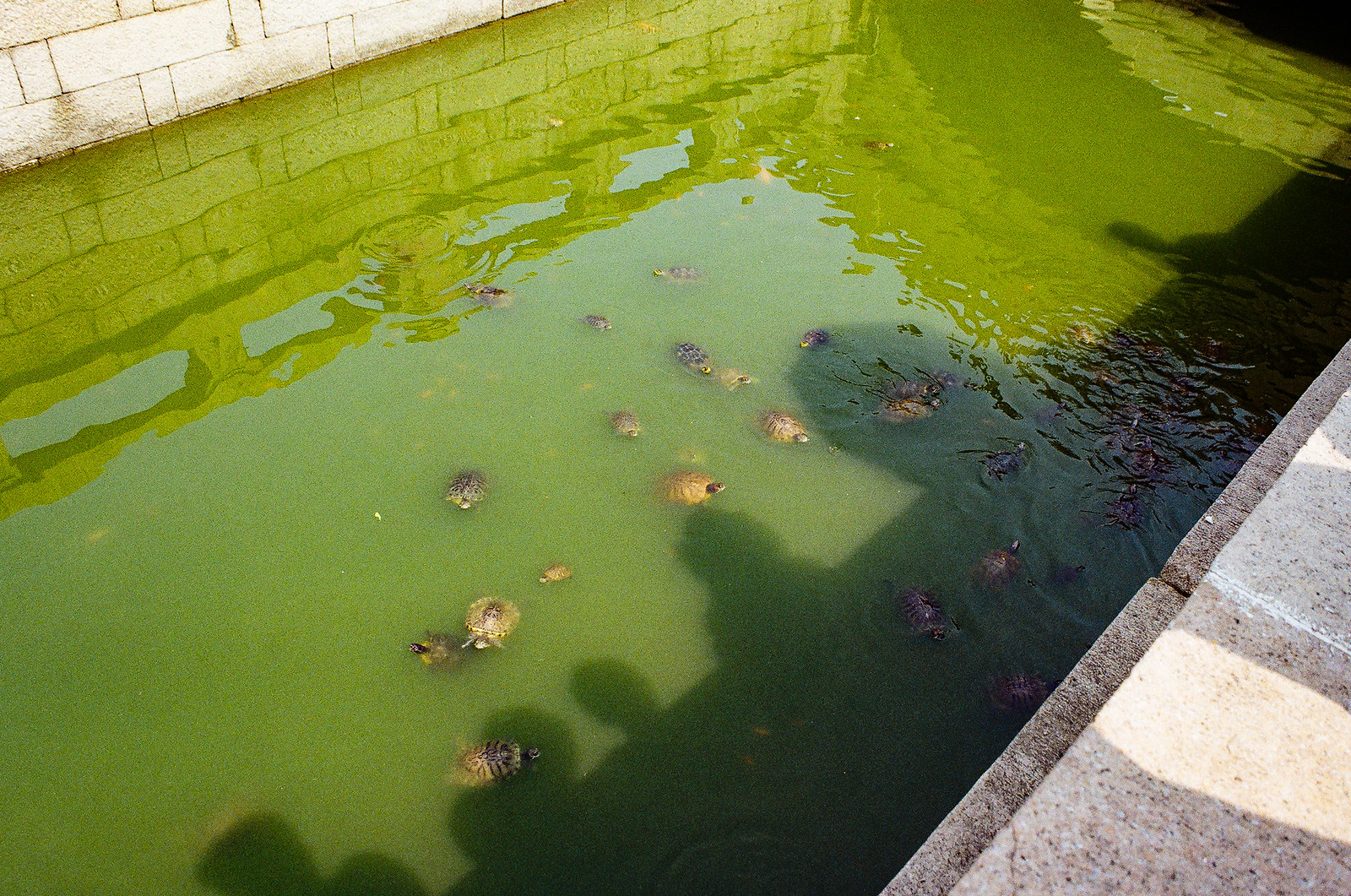This photograph captures an outdoor, sunlit enclosure housing a rectangular man-made pool constructed of stone and brick. The murky, yellow-green water, tinged with a sense of uncleanliness, contrasts against the bright daylight. Multiple turtles—some with brown and blackish shells—populate the pool, scattered across both shadowed and illuminated sections of the water. Some turtles swim closer to the wall, possibly drawn by people dropping food, while others float further out in the brighter water. The view is from a walkway above, revealing the silhouettes of several onlookers peering into the pool. A white stone wall catches the light at the top left, casting a reflection into the still water, and possibly supported by horizontally aligned pillars. The top right displays another part of the stone wall, casting a shadow that further intersects with the shapes of the observing individuals, contributing to the layering of light and shadow throughout the scene.